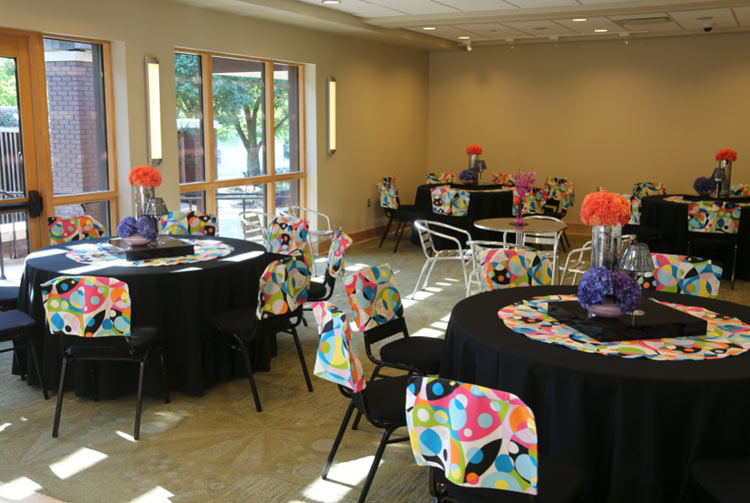The photo captures the interior of an event center, meticulously arranged for a celebration. The room features four round tables, each adorned with black tablecloths and additional colorful cloths with intricate dot and design patterns in bright shades. Six to seven black chairs encircle each table, their seat backs covered in the same vibrant, decorative fabric. At the center of each table rests a black square tray, holding two vases: a tall one and a short one, both filled with an array of purple, orange, and blue flowers. Additionally, a smaller white or silver table with a wooden top stands in the room's center, accompanied by two chairs and a small floral centerpiece. Large windows reveal a view of brick columns and surrounding trees, adding natural light to the festive setting. The overall atmosphere suggests a celebratory event, though the specific occasion remains unidentified.